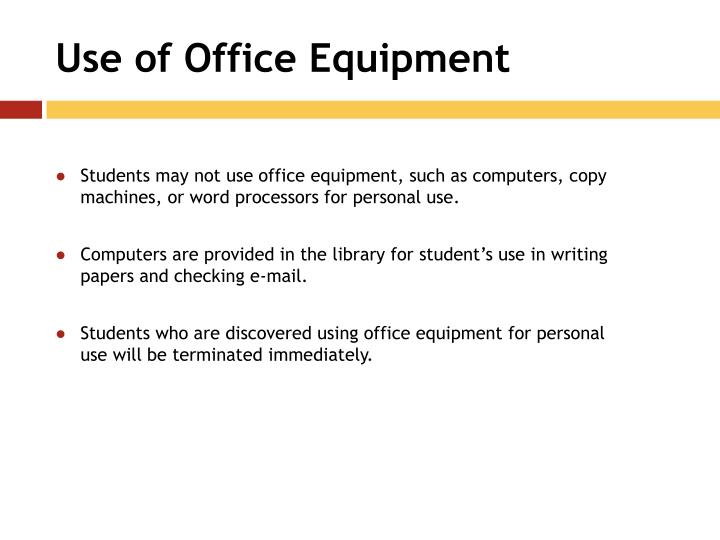The image depicts a PowerPoint slide with a white background. At the top, in bold black letters, it reads "Use of Office Equipment." Directly beneath this title is a horizontal line that resembles a pencil, featuring a small red rectangle at the far left, followed by a yellow segment. Below the line, there are three bullet points with red bullets. The first bullet point states, "Students may not use office equipment such as computers, copy machines, or word processors for personal use." The second bullet point informs, "Computers are provided in the library for students' use in writing papers and checking emails." The final bullet point warns, "Students who are discovered using office equipment for personal use will be terminated immediately." The slide outlines rules likely intended for high school or university students regarding the use of office equipment.